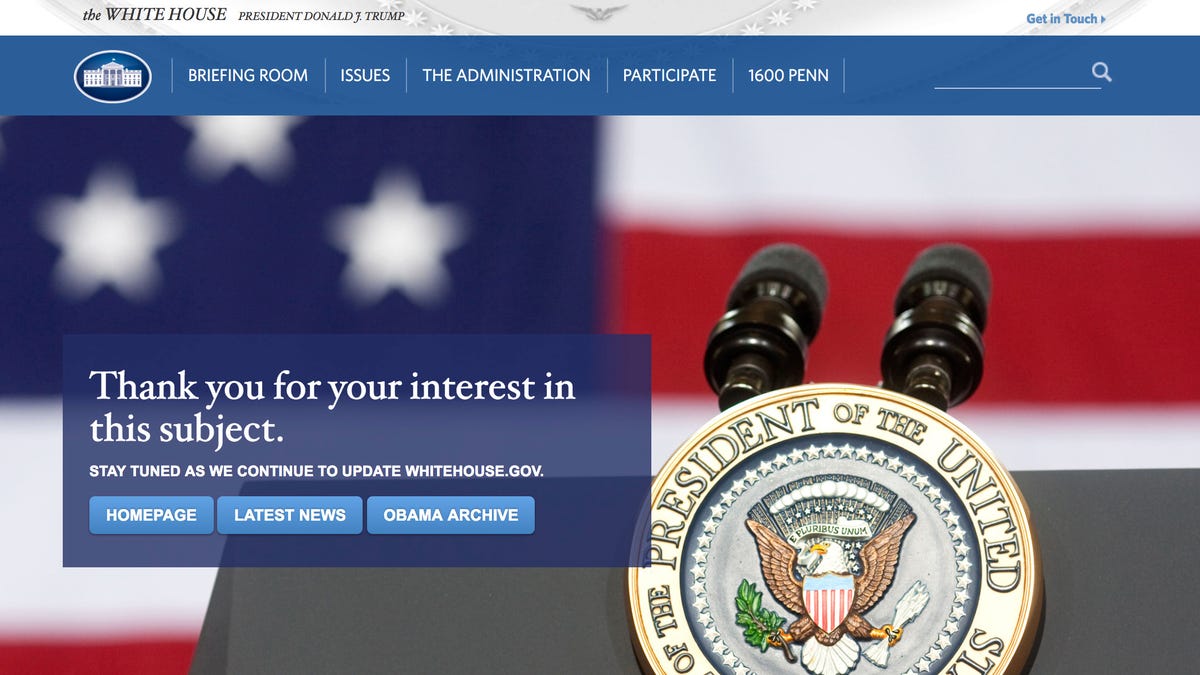The image features a webpage design with a silver bottom section and a top-left corner showcasing a depiction of the White House. Prominently displayed on the page is the name "President Donald J. Trump." Adjacent to this, there is a symbol resembling the White House. Below this symbol, a blue rectangle contains white text with the words "Briefing Room," "Issues," "Administration," "Participate," followed by "1600 Pen" and an underscore. An American flag is also visible on the page.

There is a message on the page that reads, "Thank you for your interest in this subject. Stay tuned as we continue to update WhiteHouse.com." On the right side of the image, there is a podium featuring the President's official seal—a blue circle surrounded by white stars and an eagle in the center. The background prominently includes the American flag and a mixture of white and blue squares, marked by out-of-focus stars, indicating a patriotic theme.

The webpage also presents several navigational elements, such as "Home page," "Latest news," and a section labeled "Obama Archive." The overall page appears to be part of the official White House website during President Donald J. Trump's administration, emphasizing the national symbols and official communications of the office.